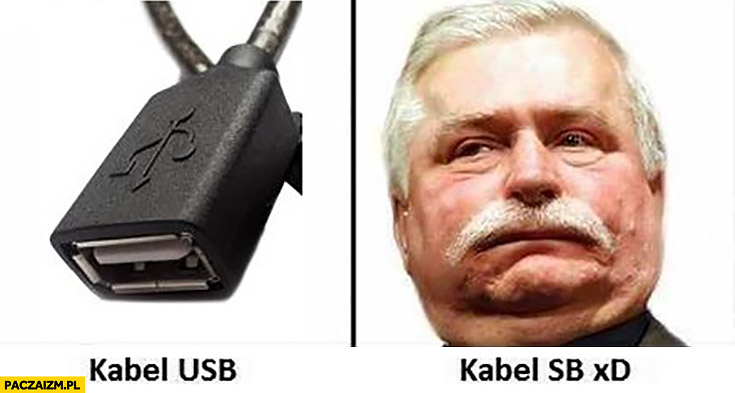The image is a rectangular meme, divided into two halves, featuring a contrast for humorous effect. On the left side, there's an image of a black USB cable with the text "KABEL USB" (using a "K" instead of the typical "C"), written underneath the opening part of the attachment. The background of this side is white with a yellow rectangle in the lower left corner that includes the black text "pakzaysm.pl," indicating a web address. On the right side, the image showcases an older white man with short, white hair and a large white mustache. His cheeks are puffed out, giving him a constipated or displeased look, with his lips tightly closed, and there are noticeable fat rolls on his chin extending into his cheeks. This side of the image has the text "KABEL SB XD," likely playing on the similar appearance of the words, with "XD" representing a laughing emoticon. Both halves are separated by a line, highlighting the humorous comparison.